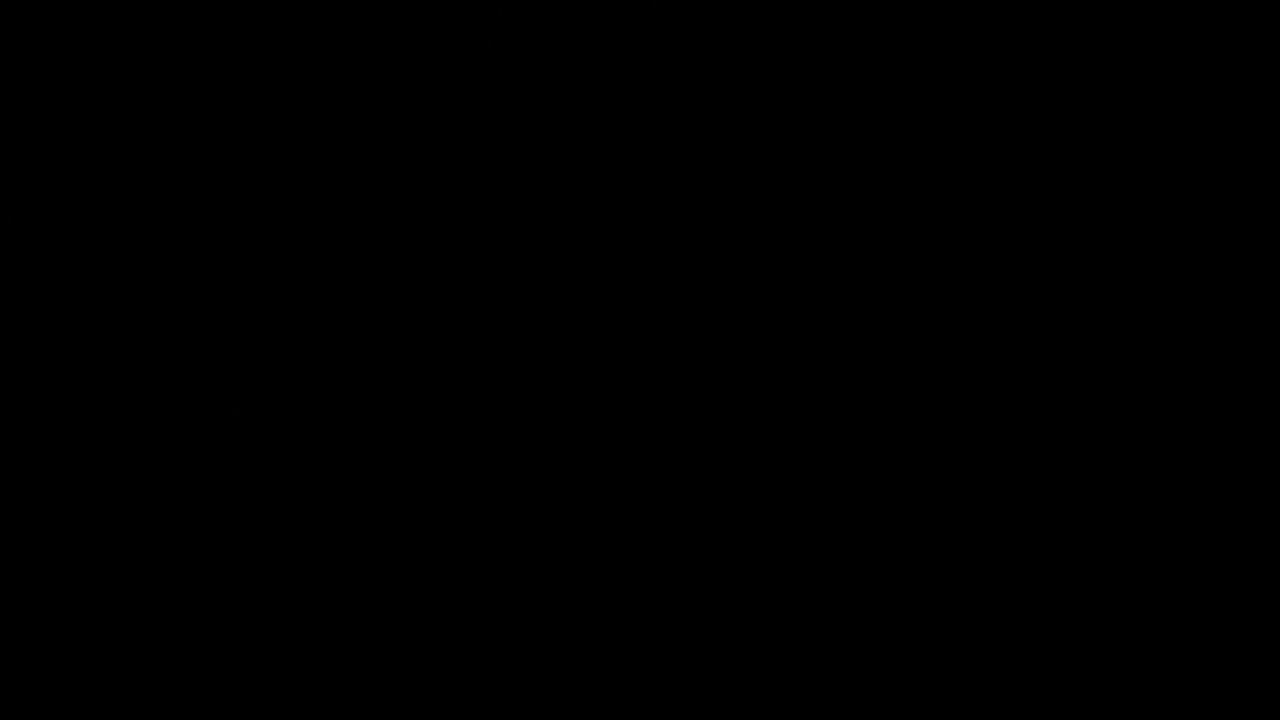The image is a plain black rectangle in landscape mode, devoid of any objects, text, or discernible setting. The background is a deep, uninterrupted black, playing tricks on the eyes and imagination with its illusion of depth; at times appearing like a void one could fall into, and at other times, seemingly reaching out. This intriguing visual phenomenon might evoke thoughts of a cinematic abyss or a malfunction, leaving the viewer to ponder its purpose. The image's dimensions are about a third wider than it is tall, further emphasizing its flat, featureless nature.